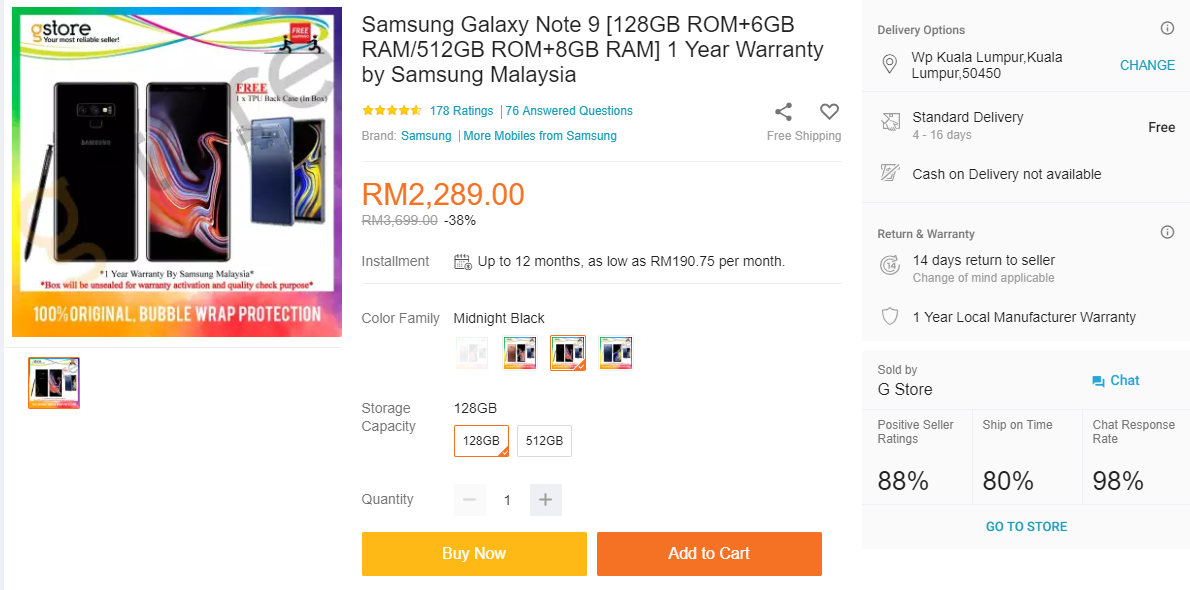Screenshot of a Malaysian E-commerce Website Listing the Samsung Galaxy Note 9

The image is a detailed screenshot of a Malaysian e-commerce website showcasing the Samsung Galaxy Note 9 for sale. The entire interface is set against a white background.

**Top Left Corner:**
- The corner displays promotional text indicating that the phone is "original, 100%" and mentions "bubble wrap protection." 
- Below this text is a smaller image of the Samsung Galaxy Note 9 on a vibrant, colorful backdrop.

**Center of the Image:**
- Prominently features details about the Samsung Galaxy Note 9:
  - Model: Samsung Galaxy Note 9
  - Storage Options: 128GB ROM with 6GB RAM / 512GB ROM with 8GB RAM
  - Warranty: One-year warranty provided by Samsung Malaysia
- The price is listed as 2,289 rupees.
- Additional information includes installment plans, color options, storage capacities, and quantity selection.
- At the bottom center, bright yellow and red buttons offer the options to "Buy Now" and "Add to Cart."

**Right-Hand Side:**
- Delivery options highlight the default address being Kuala Lumpur, with an option for the customer to change it.
  - Standard delivery timeframe: 4 to 16 days
  - Note: Cash on delivery is not available.
- Return and Warranty Information:
  - Return Policy: 14 days return to the seller, applicable for changes of mind
  - Warranty: One-year local manufacturer warranty
- Seller Information:
  - Sold by: G-Store
  - Offers a chat option in blue
  - Seller's Positive Rating: 88%
  - Ship On Time Rating: 80%
  - Chat Response Rate: 98%
- A clickable "Go to Store" button is highlighted in blue.

This entire section detailing delivery and seller options is set against a gray background.